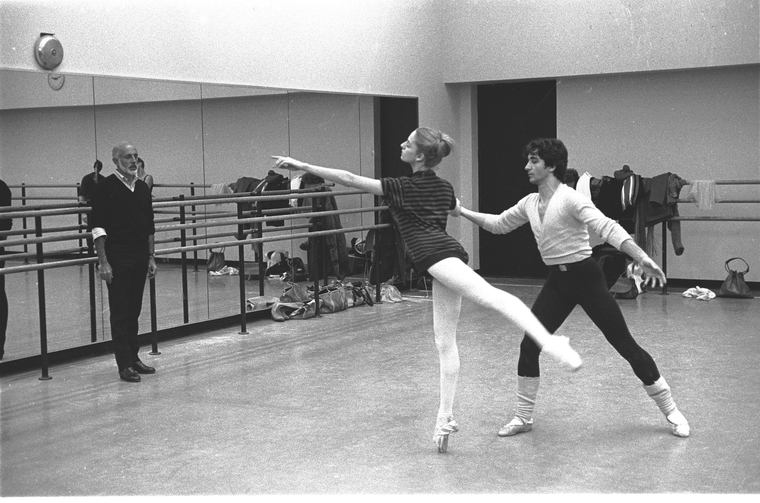In this black and white photograph taken in a ballet studio, we see a meticulously composed scene featuring three individuals. At the center of the image is a woman balancing gracefully on her right tiptoe, her left arm and leg elegantly extended. She is dressed in white tights and a short-sleeved, striped shirt, with her hair neatly tied up in a bun. To her right stands a man in a long-sleeved white shirt, black tights, and calf-high white socks. His right arm reaches forward and his left arm extends behind, giving an impression of stability and support to the woman. 

To the left of the two dancers, an older, bald man dressed in black with a lighter undershirt observes them closely, suggesting he is likely the instructor. The studio is equipped with a large mirror behind the instructor, reflecting the scene, and ballet bars are visible along the mirrored wall. The ceiling is white and features a fire bell, adding to the detailed setting of the room. Various items of clothing hang from the bars, contributing to the environment of a working dance studio. The photograph captures the disciplined and supportive atmosphere of a ballet practice in striking monochrome tones.